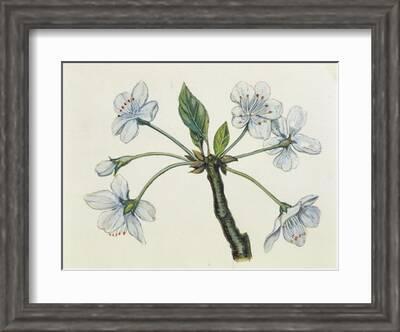This photograph features a framed botanical illustration. The frame is an olive-gray color, accompanied by a solid white mat with a bevelled edge. The illustration, set against a beige or off-white background, depicts a green stem with several green leaves at the top. Radiating from the central stem are three sub-stems on each side, each adorned with white flowers resembling orchids. The flowers are detailed, with five of the six fully bloomed, while one on the left remains tightly closed. This finely detailed illustration appears like something found in a flower guide, emphasizing the natural beauty and intricate details of the plant.